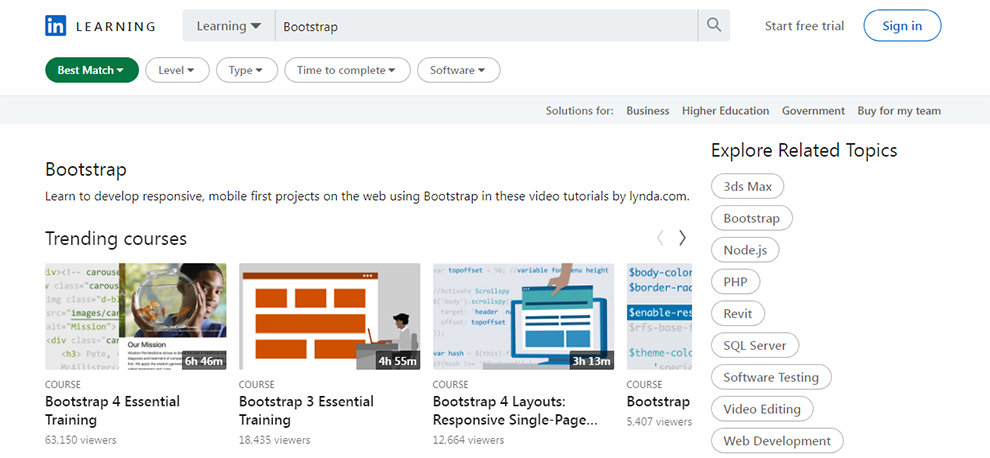This is a detailed caption for the provided screenshot of a website:

The screenshot depicts a website with a structured and clean layout. The header at the top-left corner is white and includes a small blue square containing the lowercase text "IN" in white. Adjacent to this blue square, outside its boundary, is the word "LEARNING" in all-capital dark gray text. To the right of this title, a long light gray search bar stretches across the header. On the left side of the search bar, the word "LEARNING" appears in medium gray text, followed by a downward-pointing dark gray triangle, indicating a dropdown menu. A thin medium gray vertical line separates this section from the actual search area, where the keyword "BOOTSTRAP" is entered in black text. Further to the right, after some negative space, another thin medium gray vertical line divides the search bar from a medium gray magnifying glass icon.

To the right of the search bar, dark gray text that reads "START FREE TRIAL" is visible, followed by a white button outlined in blue with blue text in the middle that reads "SIGN IN."

In the header below this layout, starting from the left, there are several pill-shaped buttons. The first is a green button with "BEST MATCH" written in white text, accompanied by a white downward-pointing triangle. Adjacent to this button are four similarly styled buttons, each white with light gray outlines and text. These buttons read, from left to right: "LEVEL" with a downward arrow, "TYPE" with a downward arrow, "TIME TO COMPLETE" with a downward arrow, and "SOFTWARE" with a downward arrow.

Beneath this row of buttons is another light gray header, with ample negative space on the left and aligned text starting towards the center of the page. This dark gray text reads, from left to right: "SOLUTIONS FOR: BUSINESS, HIGHER EDUCATION, GOVERNMENT, BUY FOR MY TEAM."

The main body of the page, which lies beneath this secondary header, has a white background, helping to maintain the webpage's overall clean and organized appearance.